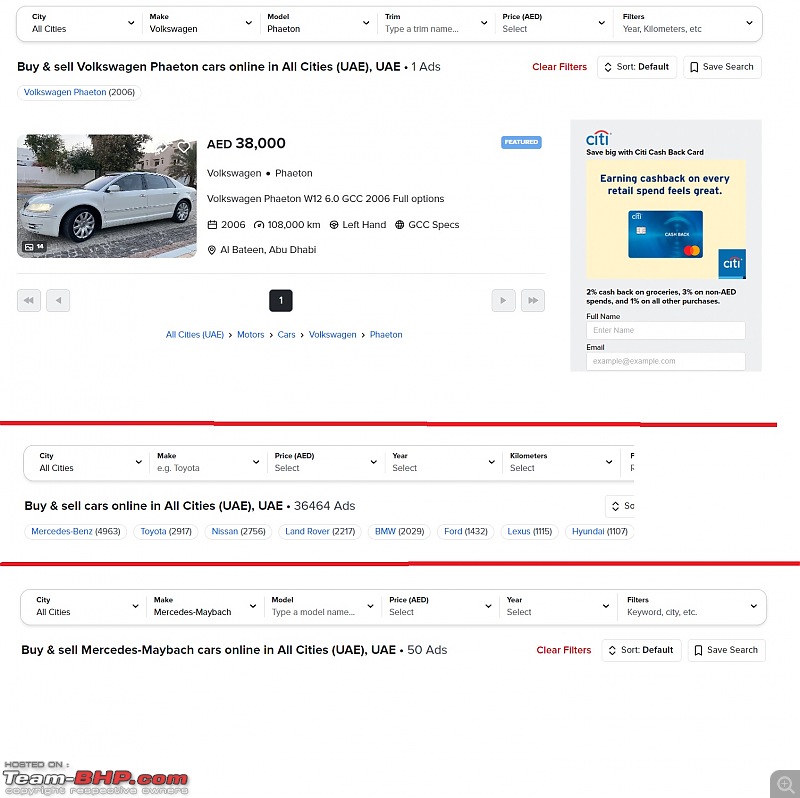A detailed website screenshot showcases a car sales platform with an extensive filtering system at the top. Drop-down menus allow users to filter by City (defaulting to "All Cities"), Make (currently set to "Volkswagen"), Model (Phaeton), and Trim (with a placeholder for Trim Name). An additional field permits price selection, displayed in AED (Arab Emirates Dirhams), along with options for further filter criteria such as Year and Kilometers.

Below the filters, a prompt reads: "Buy and Sell Volkswagen Phaeton cars online in all cities (UAE)." Adjacent to this text is an image of a white Volkswagen Phaeton listed for AED 38,000. The detailed listing specifies: "Volkswagen Phaeton W12, 6.0, GCC 2006, Full Options. 2006, 108,000 KM, Left Hand, GCC Specs." The seller is noted as "Al Bateen, Abu Dhabi," and a small black box with a number 1 is visible. A prominent red line divides sections of the webpage.

Further drop-down menus appear below the red line, with similar filtering capabilities allowing searches by City, Make, Price, Year, and Kilometers. There is also a general call-to-action: "Buy and Sell cars online in all cities," boasting a total of 36,464 ads. Specific car brands and their ad counts are listed: Mercedes-Benz (4,963), Toyota (2,917), Nissan (2,756), Land Rover (2,217), BMW (2,029), Ford (1,432), Lexus (1,115), and Hyundai (1,107).

Another red line segregates additional filtering options for the Make "Mercedes Maybach" with fields for a specific Model, Price, Year, Filters, and Keywords. The footer reiterates: "Buy and Sell Mercedes Maybach cars online in all cities." The website is credited at the bottom left as hosted on "team-bhp.com."